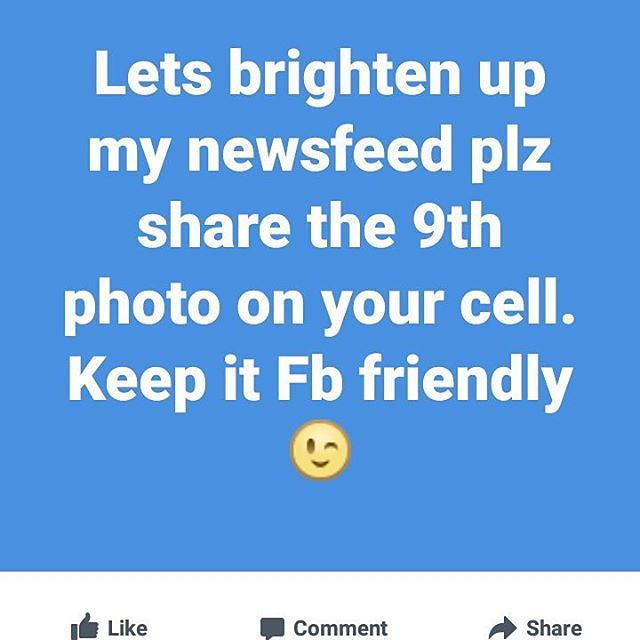The image is a Facebook post that is slightly taller than wide. The layout features a white bottom section, taking up about 10% of the image, which houses the standard Facebook like, comment, and share buttons—the thumbs up icon, speech bubble icon, and right arrow icon. The top 90% of the image has a medium to light blue background with centered white text. The text is arranged in the following lines: "Let's brighten up," "my newsfeed plz," "share the ninth photo on your cell," and "keep it FB friendly." Below this text is a winking smiley face emoji.